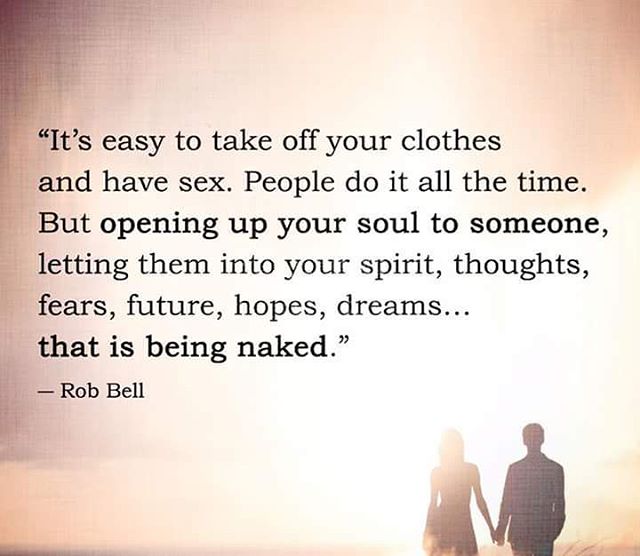The image is a computer-generated square with a visually appealing background that transitions from soft pink to a rose-colored blush, evoking the hues of a serene sunset. Dominating the sky-inspired backdrop are shades of pink, yellow, and a bright, almost white glow. In the lower right corner, the silhouette of a man and a woman, shaded completely in black, stand holding hands, their forms cut off at the thighs. Centrally placed within the image is an inspirational quote: "It's easy to take off your clothes and have sex. People do it all the time. But opening up your soul to someone, letting them into your spirit, thoughts, fears, future, hopes, dreams, that is being naked." Authored by Rob Bell, the quote is rendered in black Times New Roman font, with the phrase "opening up your soul to someone, that is being naked" emphasized in bold to draw attention. This poignant and thought-provoking message highlights the deeper aspects of emotional vulnerability in relationships.